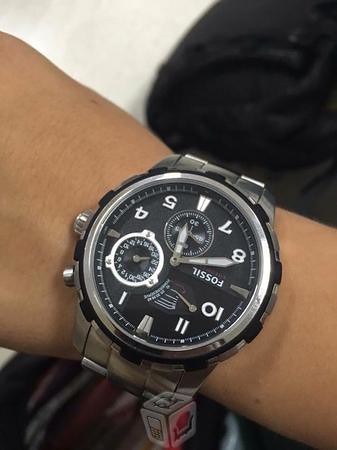This image features a close-up view of a person's wrist adorned with a large, elegant wristwatch. The individual appears to have tan skin. The wristwatch, a sophisticated timepiece by Fossil, boasts a sleek black face with bold white numerals and includes several subdials whose precise functions are unclear, although one might be for temperature tracking. The watch's band is crafted from silver and exhibits an intricate design comprising three distinct sections. At the bottom center of the image, a small gray cube-shaped logo can be seen, adorned with various symbols, including one that resembles a cell phone, among others.